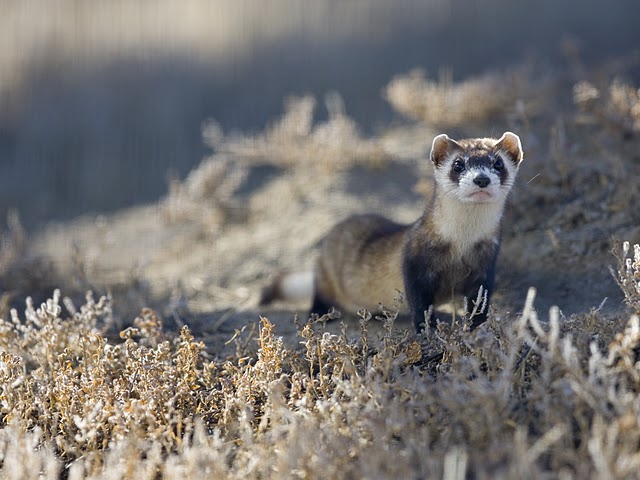The image captures a small animal in a barren, dried-out field, surrounded by withered weeds and dead plant matter. The main focus of the photo is the animal, which stands out clearly against the blurred backdrop. The creature has a slender body with brown and sable-colored fur, accentuated by a distinctive white face and chin, and a black mask around its eyes. It has short ears, a long tail, and black paws, and its pink mouth and black nose are slightly visible. The animal, possibly a ferret or a meerkat, stands alert on a dirt patch amidst the tan, brown, and white tones of the desolate environment, seemingly attentive to something in the distance.